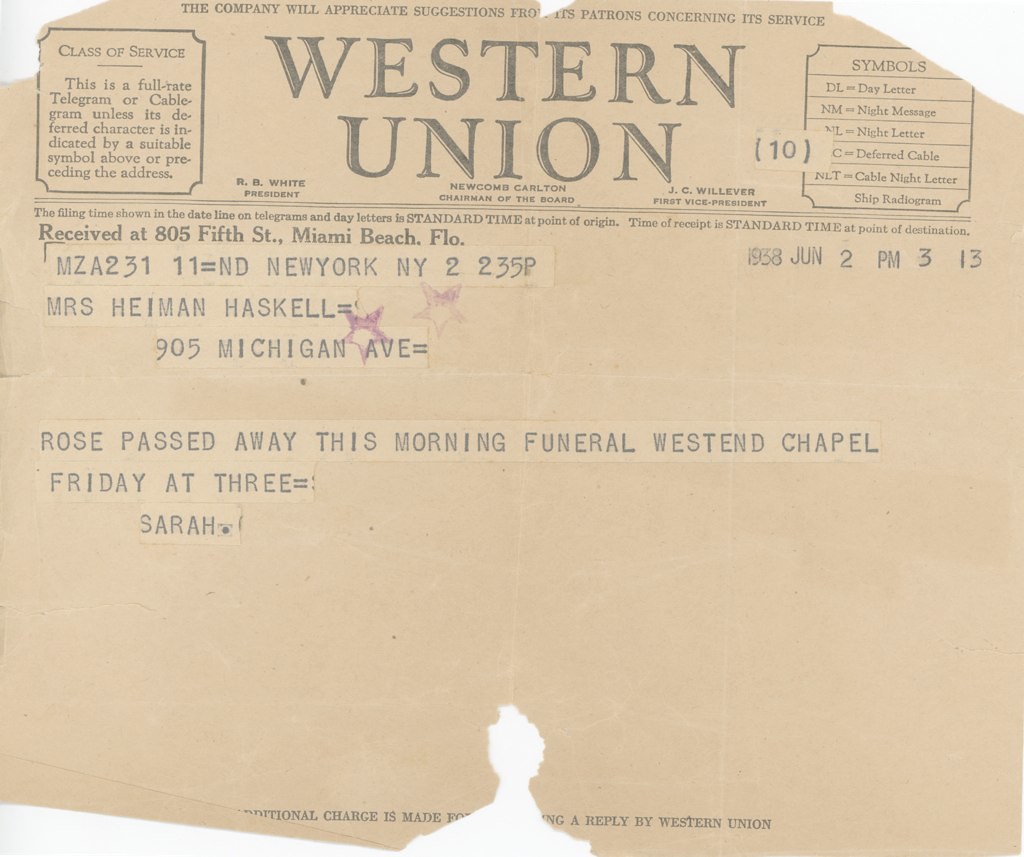This image depicts a very old and worn telegram from Western Union. The paper shows significant signs of age, with multiple tears, wrinkles, and a sandy beige color that suggests years of wear. "Western Union" is prominently displayed at the top in large, bold letters. The left corner includes a labeled box stating, "This is a full rate telegram or cablegram unless its deferred character is indicated by a suitable symbol above or preceding the address." Adjacent to this, on the right, is a list of symbols relevant to the service. The telegram contains a message in the main portion of the paper, composed of cut-out and pasted sections, detailing the sad news of a person named Rose passing away with the message: "Rose passed away this morning. Funeral West End Chapel Friday at 3, Sarah." Additional text specifies that it was received at 805 5th Street, Miami Beach, Florida, on June 2, 1938, at 2:13 PM. The address of the recipient is Mrs. Hyman Haskell, 905 Michigan Avenue, and parts of the telegram are notably torn at the bottom middle and the top corners.